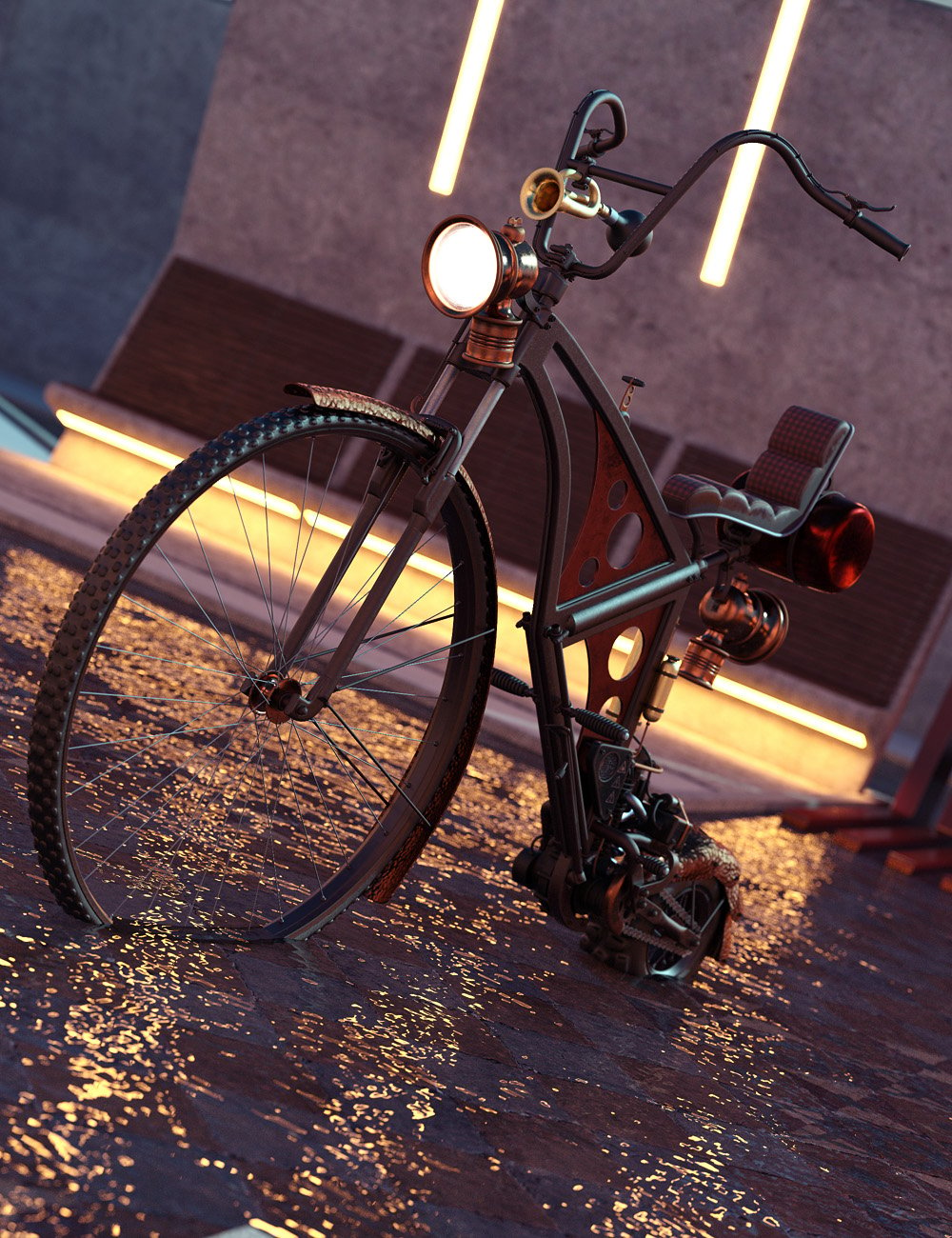The image is an artistic piece depicting an unusually designed bicycle that appears almost AI-generated due to its peculiar features and amalgamation of shapes. The bicycle has a large front wheel and a very small, training wheel-sized back wheel. The seat is minuscule, seemingly impractical for use, while the color of the bike is predominantly black. Mounted at the front of the bicycle is a large, antique-looking lantern, complemented by a toy horn situated just below the handlebars. The bicycle is placed on a surface that looks like wet pavement or shallow water, giving the impression that it is slightly submerged. The background features a grey wall and two striped lights hanging from the top, adding to the surreal and unusual atmosphere of the scene.